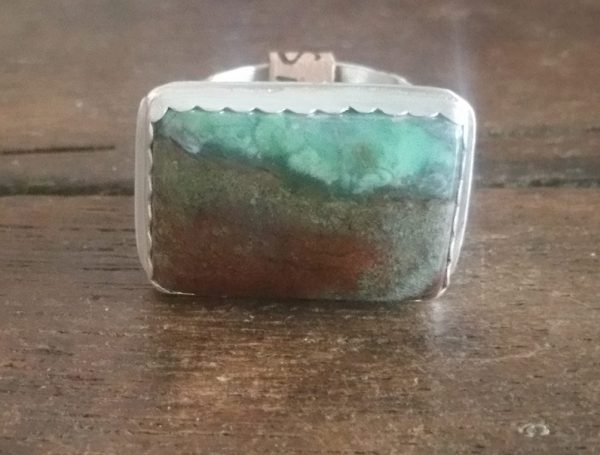The color image showcases a close-up of a handmade piece of jewelry, likely a ring, resting on an old, worn, dark brown wooden table with a visible wood grain. The focal point of the jewelry is a large, rectangular, multi-colored stone encased in a silver setting with scalloped, wave-like edges. The stone features a gradient of colors, transitioning from a jade green at the top, through a greenish-gray in the middle, to a brick-red at the bottom. The ring appears to be lying on its side, with a tag wrapped around the band, where the letters "S" and "I" can be seen. The detailed craftsmanship and vibrant colors make the piece of jewelry stand out against the rustic wooden surface.